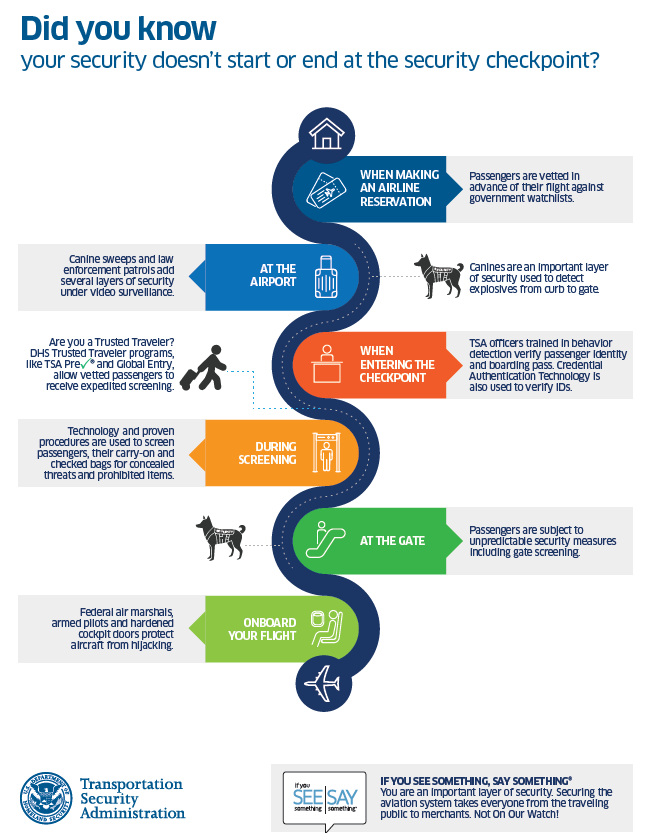This detailed TSA informational poster, set against a white background, is designed to educate travelers about the comprehensive security process. At the top, in blue text, it reads, "Did you know your security doesn't start or end at the security checkpoint?" The poster features a blue winding path that visually maps out the journey from a house to an airplane, representing the various stages of travel. 

Key steps are delineated in rectangles and annotated with clip art images including tickets, luggage, a security checkpoint, an escalator, and a person seated on an airplane. Throughout the path, informative text details each stage:

1. **Making an Airline Reservation:** Passengers are vetted against government watch lists.
2. **At the Airport:** Security layers include canine sweeps, law enforcement patrols, and video surveillance to detect explosives, represented by a dog icon.
3. **Entering the Checkpoint:** TSA officers trained in behavior detection verify identities and boarding passes. Technologies like the Credential Authentication Tool enhance security.
4. **Trusted Traveler Programs:** Programs such as TSA PreCheck and Global Entry offer expedited screening for vetted passengers.
5. **During Screening:** Proven procedures and technology are used to screen passengers, carry-on items, and check-in bags for concealed threats and prohibited items.
6. **At the Gate:** Passengers may face unpredictable security measures, including gate screening.
7. **Onboard the Flight:** Federal air marshals, armed pilots, and hardened cockpit doors protect aircraft from hijacking.

In the bottom left corner, the poster features the TSA logo, while the bottom right corner includes the message, "If you see something, say something," underlining everyone’s role in securing the aviation system.